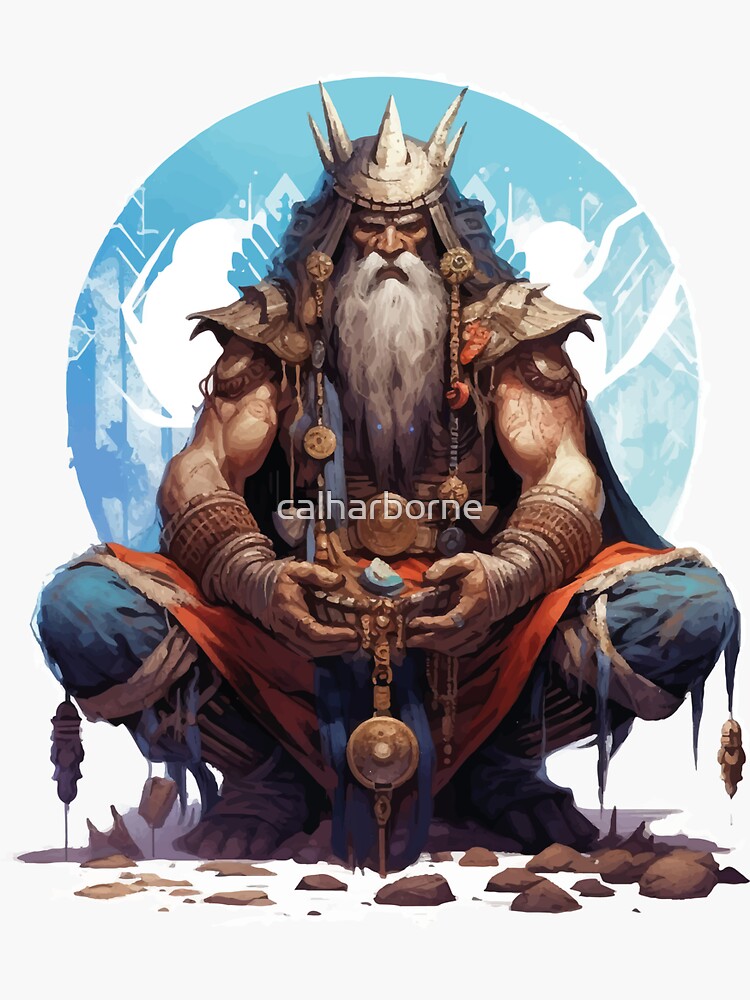This detailed illustration titled "Waterbark" by Cal Harbourn depicts a remarkably muscular, elderly warrior with a distinctive Viking appearance, squatting with intense purpose. The warrior, who is squatting with his elbows resting on his knees, clasps a valuable item wrapped in golden details. His strikingly long white beard and mustache extend down to his belly button, complementing his aged and war-weary visage. He dons a battle-worn Viking helmet adorned with five prominent spikes and ornate jewelry that dangles from its sides, featuring intricate gold emblems. His shoulder armor is wooden, and his muscular arms are bare except for cloth wraps around his wrists and hands. His attire includes blue pants paired with an orange apron-like cloth, and his bare, rugged feet rest on rocky ground. Surrounding him is a large, snow globe-shaped emblem with a light blue hue and white designs, set against a pristine white background. This visually arresting digital painting encapsulates a blend of strength, age, and fantasy warrior elements, meticulously rendered in striking detail.